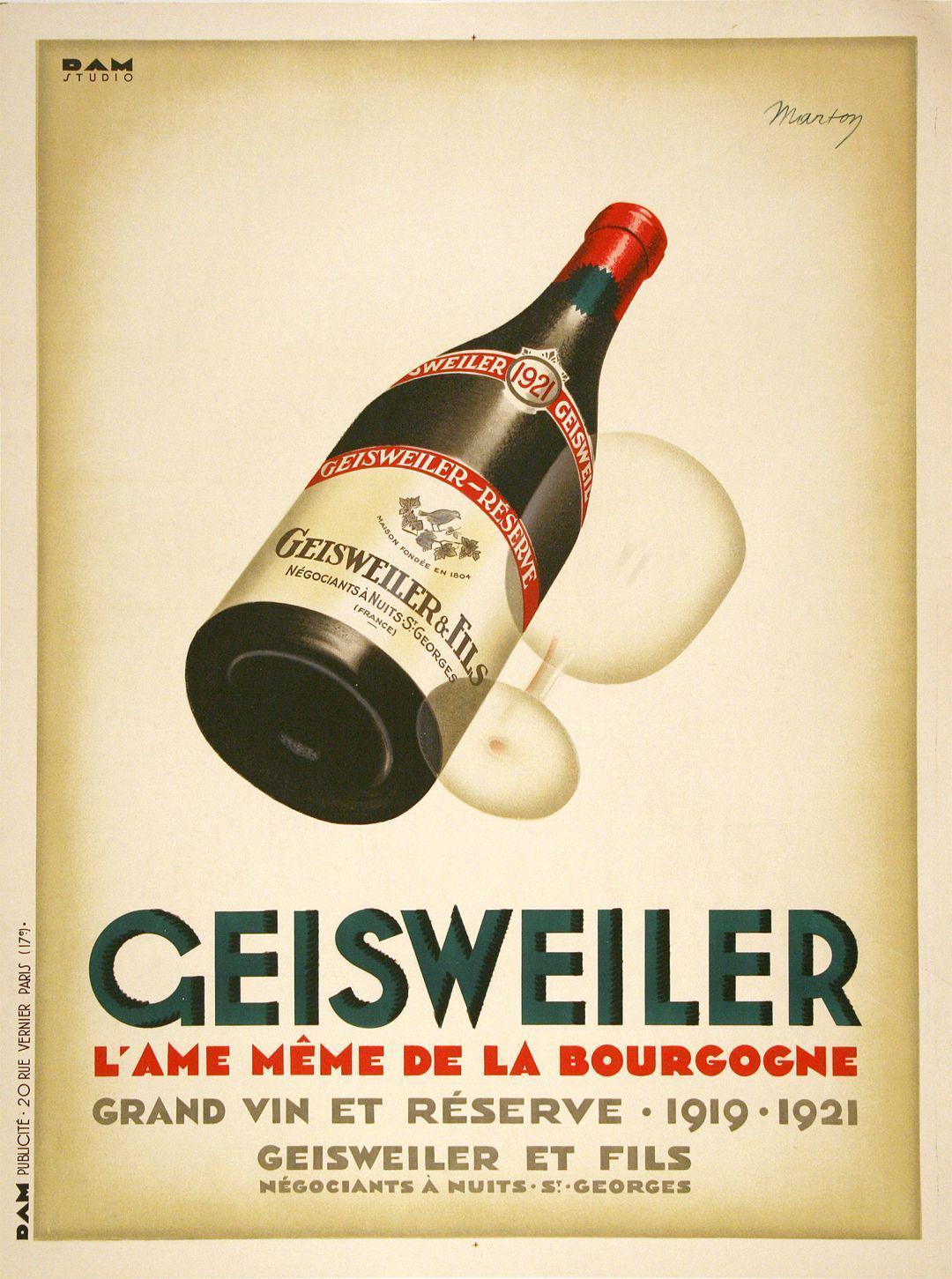The image depicts a vintage promotional poster for Geisweiler wine in a color illustration with a portrait orientation. The background features a beige gradient, darker at the edges and lighter in the center, giving it an aged look. Dominating the upper two-thirds of the image is a prominently displayed wine bottle, positioned at an angle as if viewed from below through a glass table. 

The bottle itself has distinct characteristics with a red wax cap and neck accentuated by a gold ellipse with the year "1921" and the text "Geisweiler." Below this is a cream-colored label with a red banner at the top, displaying "Geisweiler Reserve" in cream text. The central part of the label features an illustration of a bird perched on a flowery branch, adding a touch of elegance and nature to the design. At the bottom of the label, in bold black text, reads "Geisweiler et Fils."

Accompanying the bottle is a translucent wine glass positioned beside it, enhancing the promotional appeal. At the top right of the image, the name "Martin" appears in blue pen. The text on the poster includes elements in French, such as "L'Aime M'Aime de la Bourgogne," suggestive of the wine's prestigious origin, with "Grand Venet Reserve 1919 to 1921" written in red text. The overall design and detailed typography underscore the luxurious and historic essence of the Geisweiler wine.